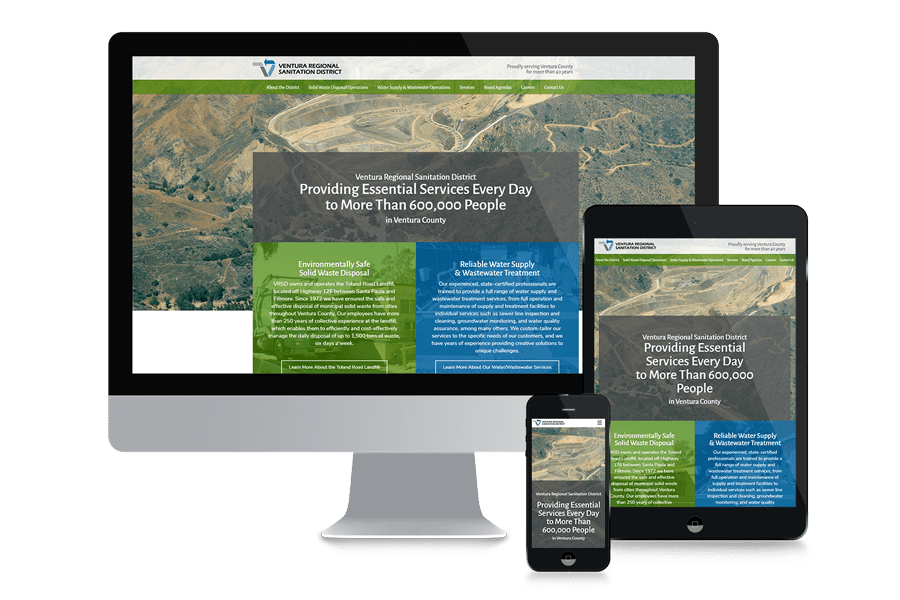The image depicts three electronic devices each displaying a visual presentation from the Ventura Regional Sanitation District. 

- The central device is a computer monitor, illustrating a comprehensive graphic that highlights the provision of essential services to over 600,000 people daily. The presentation is visually segmented with a blue section focused on water supply, and a green section emphasizing environmental services. A large map dominates the screen alongside what appears to be significant earthwork operations, possibly a sand pit, extraction site, or water management facility.

- To the left, a tablet shows a condensed version of the same graphic, maintaining the three core messages presented: water supply (blue section), environmental protection (green section), and an illustration of the earthworks.

- On the right, a mobile phone displays a much smaller and more focused image of the earthwork operations, which might be related to sewage works or water extraction facilities, though the exact nature is indistinct.

Each device encapsulates a different level of detail from the Ventura Regional Sanitation District’s visual communication, providing varying degrees of information and emphasis.